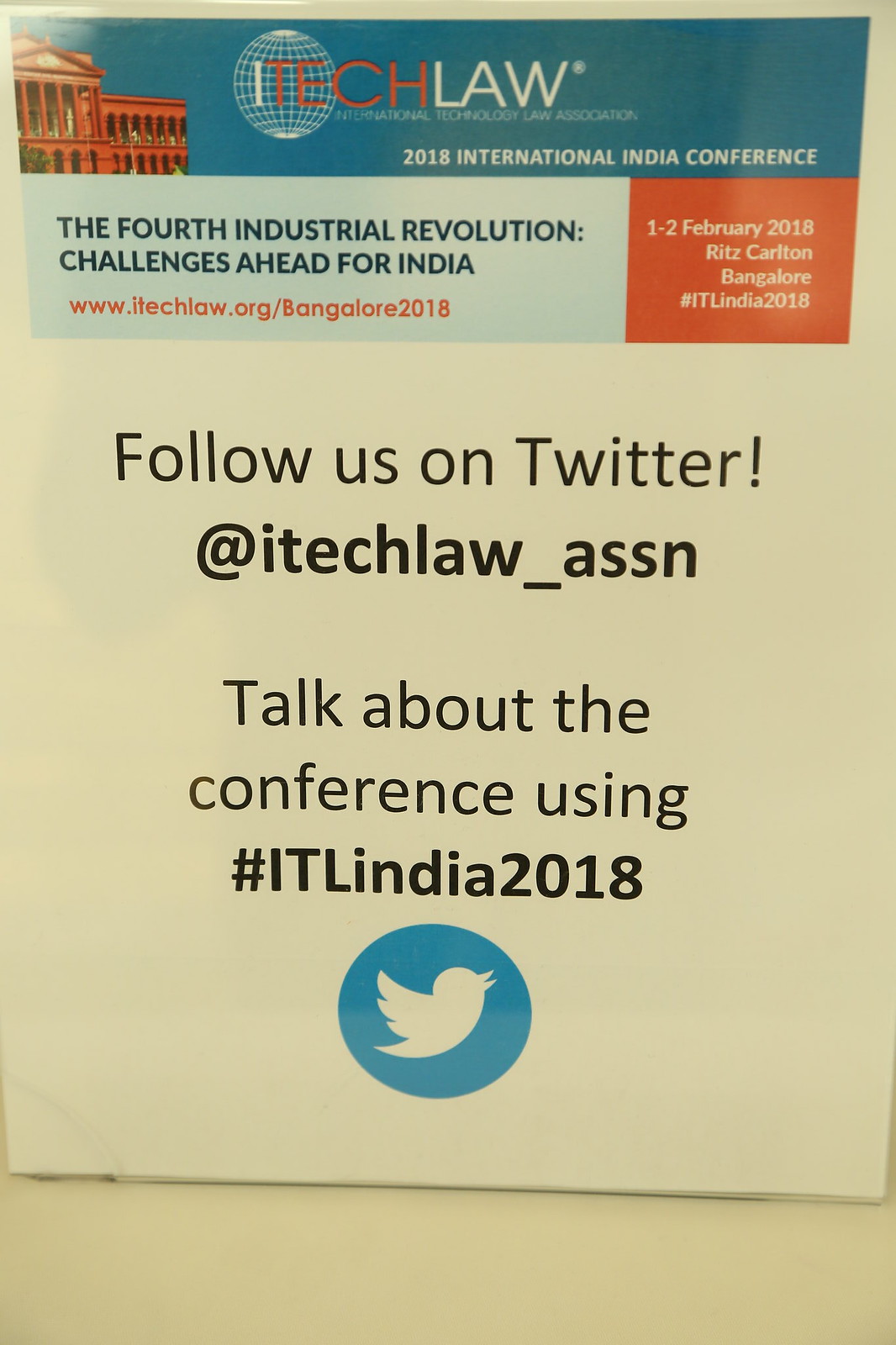The image is a detailed, color graphic design promotional flyer for iTechLaw, prominently displayed on a white painted wall. The flyer is primarily white and portrait in orientation, featuring colorful, horizontal banners across the top. The topmost banner features a red brick building with columns on the left side, leading into a solid light blue background. Centered within this banner, the logo reads "iTechLaw," with "Tech" in blue and the surrounding text in white. Behind the "ITE" and "iTechLaw" text, there is a grid-lined globe, indicating the global reach of the organization. Below the logo, in white font, it states "International Technology Law Association," and on the bottom right, the banner mentions the "2018 International India Conference."

Below this section is another light blue stripe with an orange accent on the right, highlighting the theme "The Fourth Industrial Revolution: Challenges Ahead for India." The banner includes the event details: "1-2 February 2018 at the Ritz-Carlton, Bangalore" and the URL "www.itechlaw.org/Bangalore2018." Additionally, the flyer emphasizes social media engagement, urging viewers to "Follow us on Twitter!" at @itechlaw_assn and to discuss the conference using the hashtag #ITLindia2018. The bottom of the flyer also features the blue circle Twitter logo, reinforcing the call for online interaction. The overall style is professional graphic design, effectively advertising the upcoming conference.